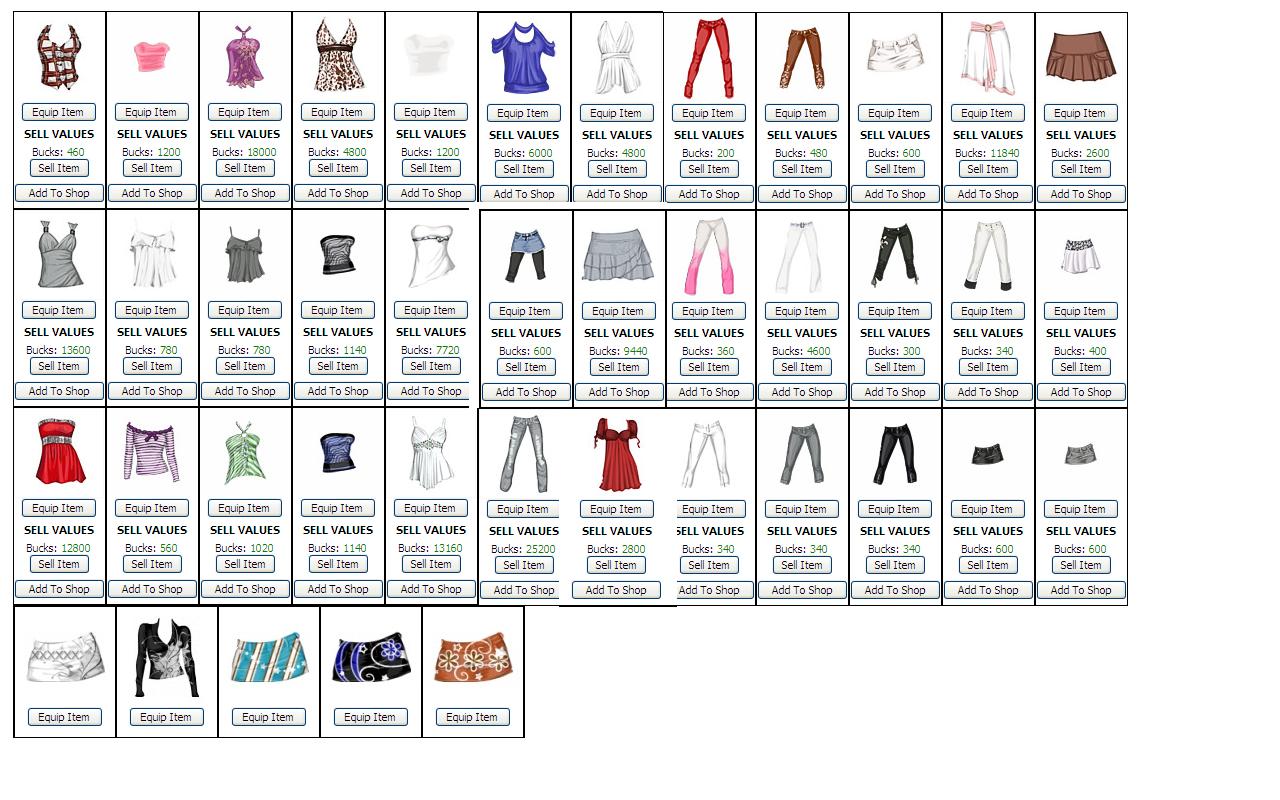The screen grab showcases an organized grid of various pieces of clothing available in a video game, set against a white background for high clarity and color contrast. Arranged in four rows, the first three rows contain 12 items each, while the bottom row holds five items, making a total of 41 distinct clothing pieces. Each item is neatly displayed within its own rectangle.

Starting from the top left, the first item is a white and red plaid sleeveless tank top with buttons, followed by a pink crop top with short sleeves to its right. The garments range across different categories, including tops, bottoms, skirts, and dresses, displayed in various colors such as pink, red, brown, white, purple, and green.

Under each clothing image, there is a consistent layout of interactive buttons. From top to bottom, the options include an "equip item" button, followed by the "sell values" displaying sell prices (for example, $4.50 or $4.60), a "sell item" button, and finally an "add to shop" button. The clarity and quality of the image are excellent, with all words and buttons clearly visible, ensuring an easy and detailed browsing experience for the user.